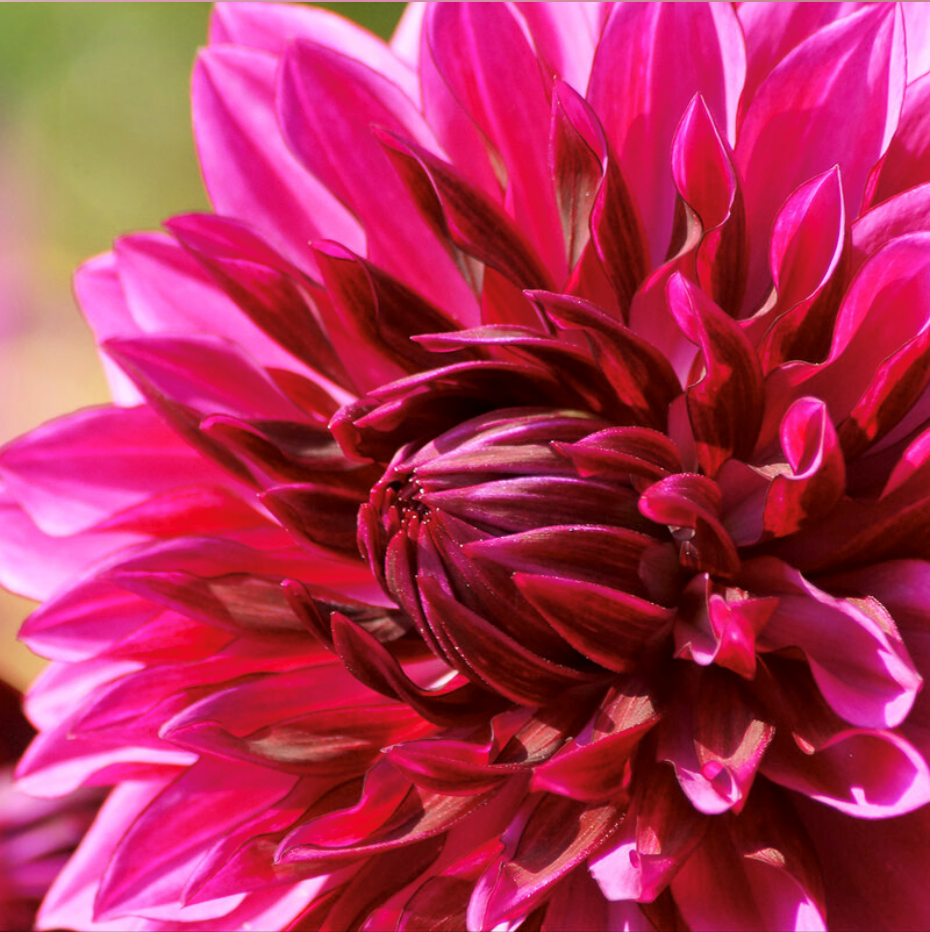This vibrant and detailed image captures a large, blooming flower rendered in brilliant shades of pink, purple, and red, with a stunning, sunlit reflection enhancing its radiance. The flower's outer petals have spread wide, displaying lighter hues that border on white, glistening with sunlight. The core of the flower, which faces diagonally to the left, remains in the process of blooming, showing a stark contrast as it transitions from a curled-up dark red center to the gradually lightening partially-bloomed layers. The high-resolution or close-up perspective suggests the flower might be immense in size, perhaps an optical illusion created by the photo's framing, dominating the foreground against a softly blurred, green grassy background hinting at a garden setting. The interplay of colors and the ongoing bloom process is the central focus here, highlighting the flower's striking beauty and intricate details.